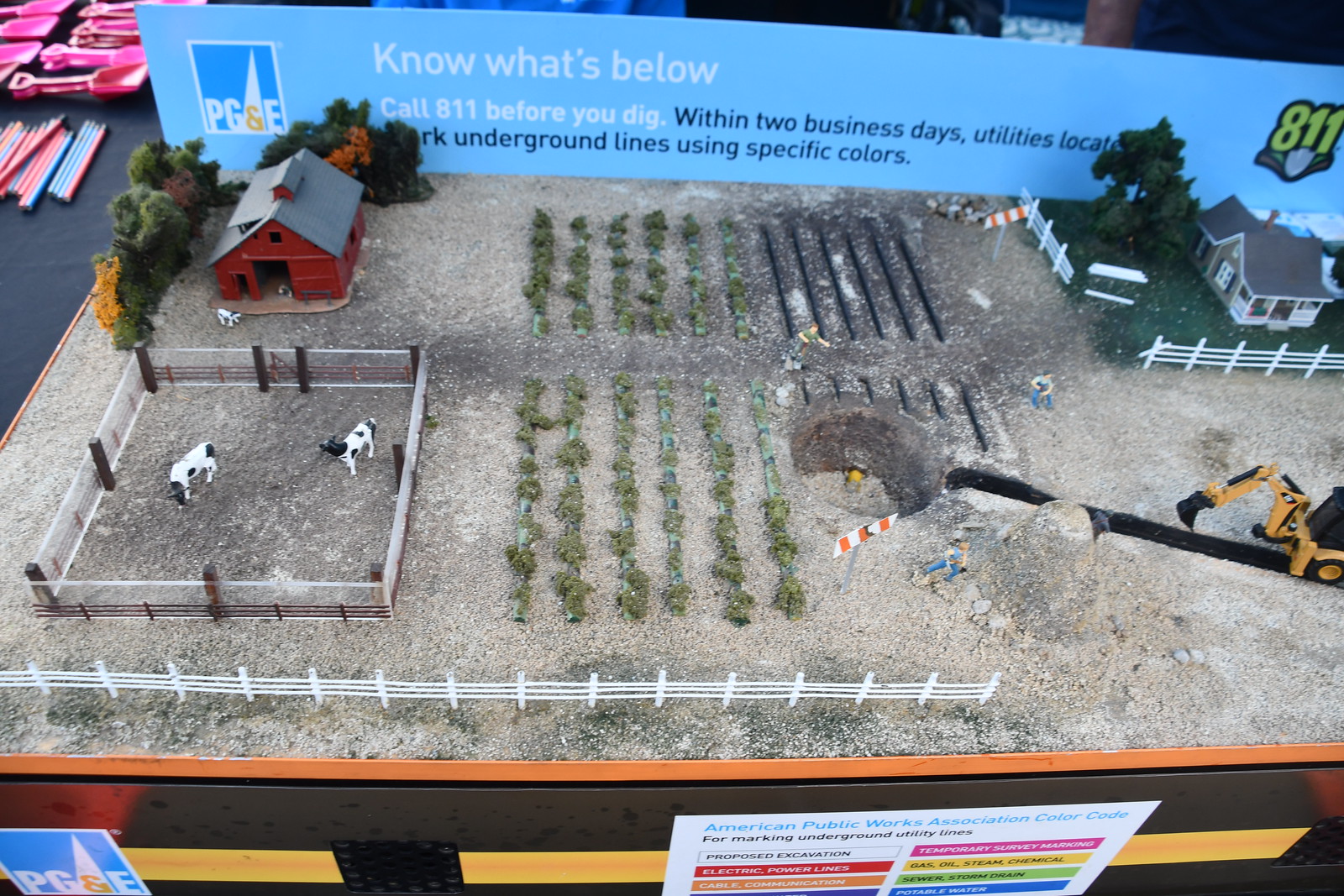The image showcases a detailed photograph of a diorama depicting a miniature farm, used as an advertisement for a display or table. The background is a solid blue with the text "Know what's below. Call 8-1-1 before you dig. Within two business days, utilities locate underground lines using specific colors." 

In the diorama, on the left side, there's a white corral with two toy black and white cows. Behind the corral, a small red barn with a gray roof stands surrounded by trees. The central part of the diorama features several green rows of vegetables representing farm fields. Towards the center right of the image, a large circular pit with a trench and a yellow construction truck, possibly a crane, can be seen, indicating some sort of construction, perhaps digging a well. Near this, at the bottom right, there's a caterpillar tractor or earth mover. 

On the upper right corner of the diorama, a one-story house with olive-colored walls, white siding, window sills, and a gray roof sits behind a broken white picket fence. There are trees and patches of green grass surrounding the house, suggesting it’s the farmer's residence. The entire scene is viewed from a top-down perspective, capturing the essence of a well-detailed farm setup.